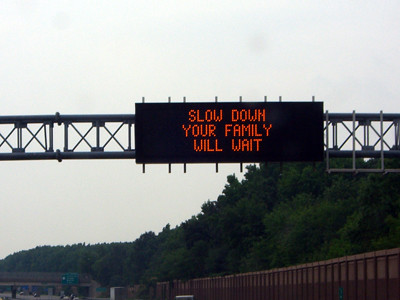This daytime color photograph captures a highway scene under a hazy, overcast sky with a light bluish-gray tint. The focal point of the image is a rectangular, black digital road sign centered on a metal girder that spans the entire width of the road. The girder consists of two horizontal poles connected by evenly spaced X trusses. The electronic sign displays the cautionary message "SLOW DOWN, YOUR FAMILY WILL WAIT" in vivid orange, capital letters. Below the girder, slightly to the right, a row of tall trees in varying shades of light and dark green lines the roadway. In the distant background to the left, hills densely covered with more trees create a sense of depth, while faintly seen road barriers and a few vehicles, including at least one truck, indicate that we are on a busy highway.